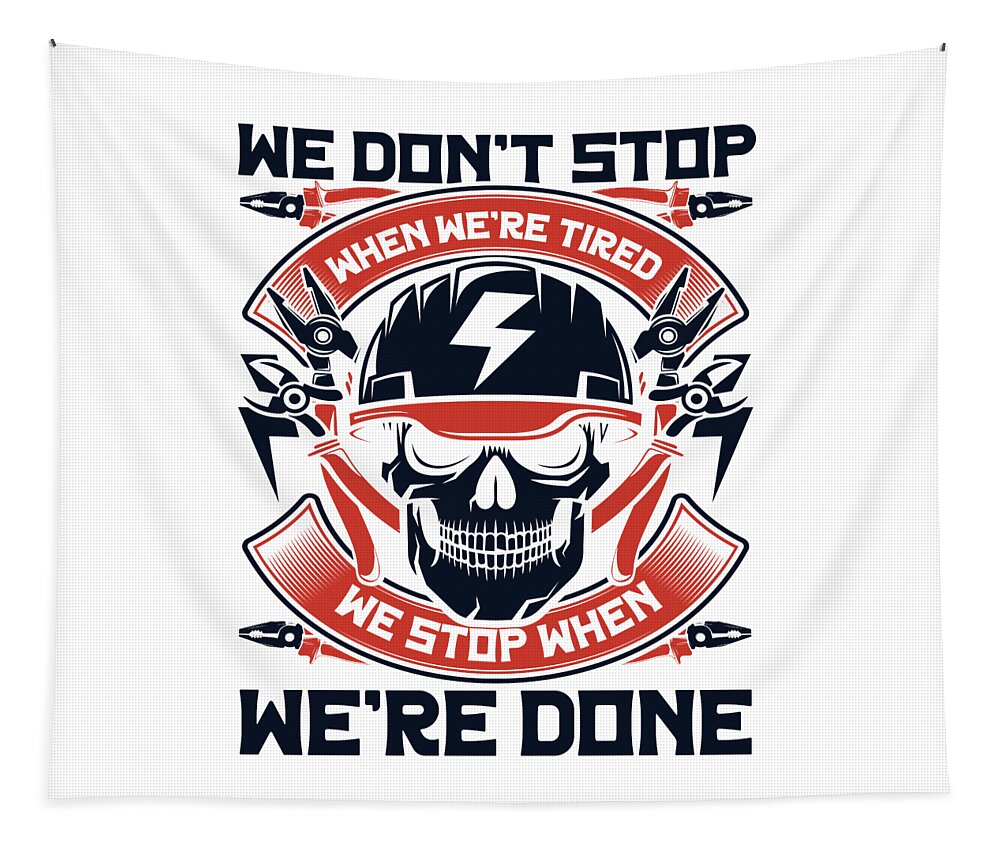This image depicts a square banner made of textured white fabric, secured to a wall by stick pins at its top right, left, and corners. Dominating the center is a black skeleton adorned with a black helmet that features a prominent white lightning bolt and a red brim, accented with red cords on either side. Flanking the skeleton, both to the left and right, are illustrations of tools such as pliers and wire cutters. Across the top of the banner, in bold black text, it reads, "We don't stop." Below, in red text enclosed within an arching banner, a continuation of the slogan declares, "When we're tired, we stop when we're done." This eye-catching piece, with its limited color palette of black, red, and white, appears to promote a diligent, unwavering work ethic, possibly associated with an electrical contracting company or a specialized unit, as suggested by its imagery and slogans.